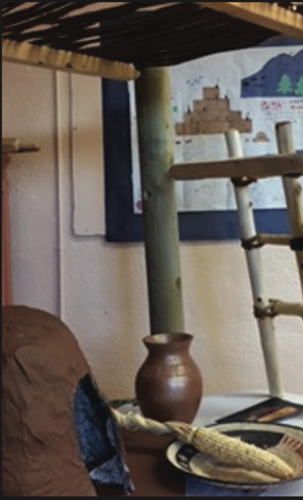The image depicts an indoor scene with a rustic, earthy aesthetic. At the center, there is a long pole supporting a roof-like structure, which casts a cozy ambiance over a table beneath it. On the table sits a pottery-style vase with a rich brown hue, exuding an old-world charm. To the right of the vase is a white plate with ornate curved edges; the plate holds cobs of corn still in their husks, suggesting a farm-to-table theme. The background features a wall adorned with a quilted art piece that has a dark blue border and intricate appliqué designs resembling mountains and trees. The wall is also interrupted by small pipes or wiring. Resting against the pole is a wooden ladder, adding to the room's rustic feel. The setting is subtly lit, possibly by natural light filtering from an unseen source, enhancing the textured details of the exposed wiring and the layered wall hanging.